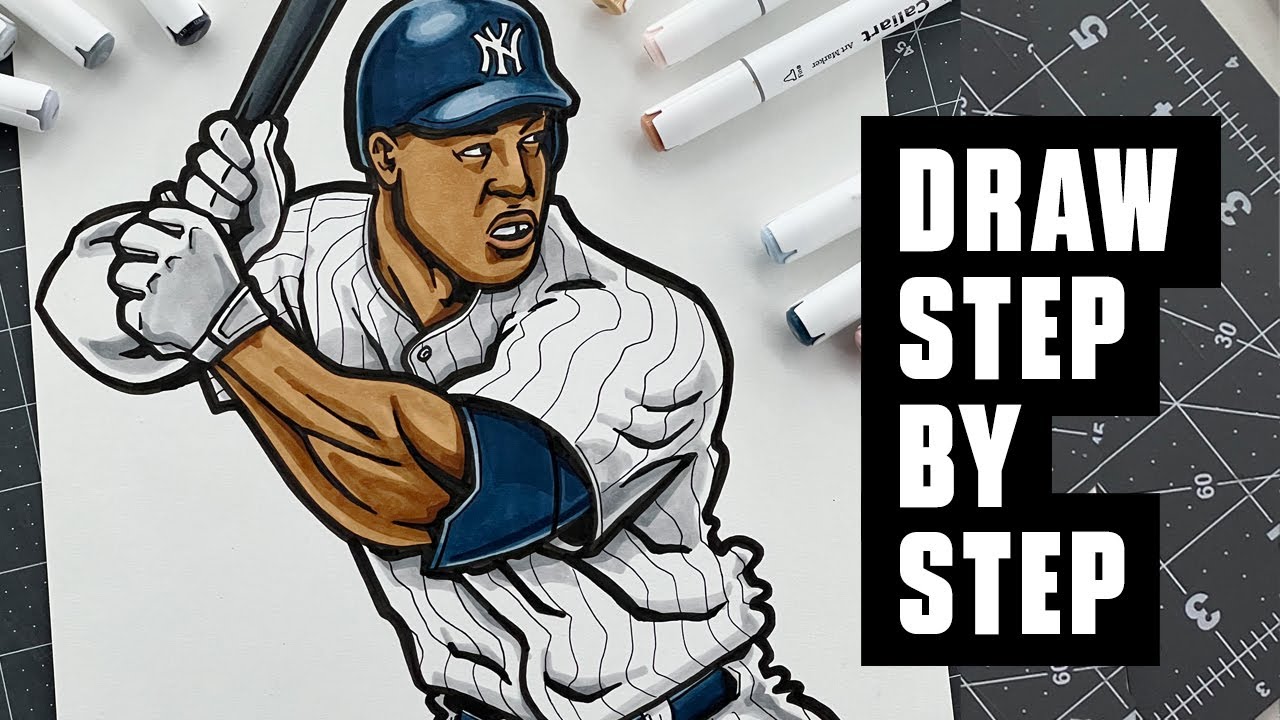This image, clearly intended for a tutorial, features an intricately detailed drawing of a New York Yankees player on a white piece of paper. The paper, situated on a numbered gray drafting mat, is surrounded by white markers with various colored tips such as black, blue, brown, pink, and beige. The player, depicted with brown skin, has a gap in his teeth, big muscular arms, and is donned in a classic Yankees pinstripe uniform. He wears white gloves, and a blue undershirt is visible peeking from his right sleeve, complemented by a blue belt. His helmet bears the iconic New York Yankees symbol, and he grips a black bat as though ready to hit. To the right, large white text on a black background boldly states "Draw Step-by-Step," making it clear that this is a step-by-step drawing tutorial.